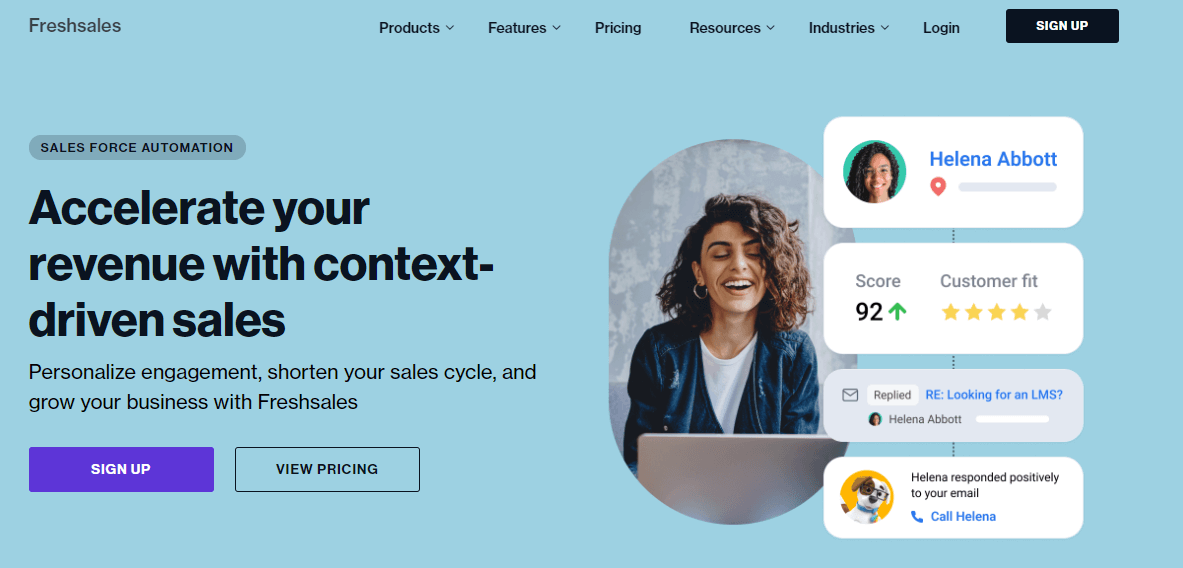Discover FreshSales: 

Transform your sales approach with FreshSales by leveraging advanced sales automation to accelerate revenue. With context-driven tools, you can personalize engagement, shorten the sales cycle, and drive business growth. Explore features, pricing options, and resources tailored to various industries by visiting our website. Log in or sign up to get started. Experience seamless integration with services like Salesforce and enjoy a streamlined process for managing your sales pipeline. Whether you're looking to enhance email outreach or improve call management, FreshSales provides the solutions you need. Visit us today to view pricing and sign up for a demo. Feel free to leave your comments and feedback.